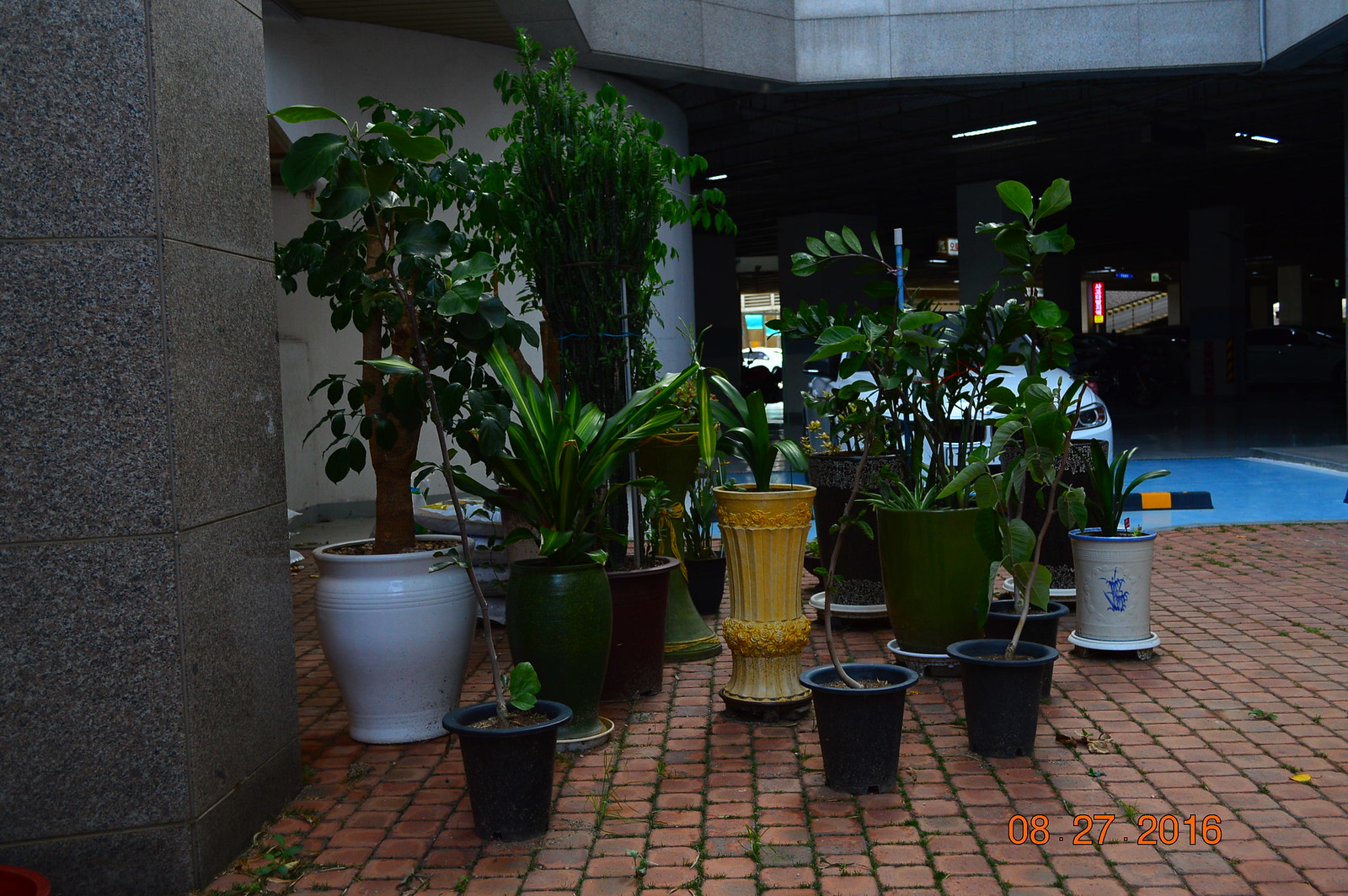The photograph, taken on August 27, 2016, as indicated by the orange date imprint on the bottom right, depicts an outdoor area that appears to be part of a hotel or parking structure. The ground is paved with square brick tiles, some of which have green moss growing between them. A variety of potted plants, totaling twelve and ranging in size, are prominently featured in the foreground; these include small leafy plants, snake plants, and several trees with thin trunks and lush green leaves. The plants are set around a white vehicle that is parked on the left of the image near a concrete or marble pillar.

Additionally, there is a concrete block colored in orange and black visible on the ground, and in the background, there's a mix of architectural elements— including a passageway or doorway, more pillars, and black-and-yellow lined structures, suggesting it's near or part of a parking area. An illuminated red-and-yellow sign and another parked car are faintly visible in the dimly lit background, which also shows a hint of stairs leading to other parts of the building. The detailed setup of the scene, with the combination of structures, vehicles, and diverse plants, creates an intricate and well-preserved environment.